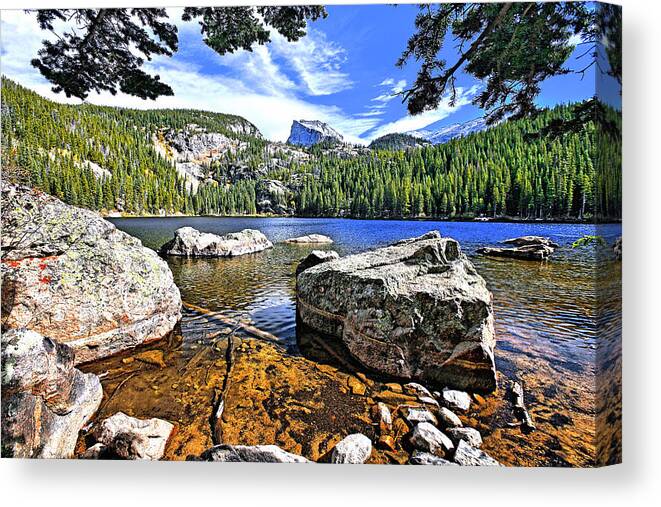The image depicts a detailed and serene landscape with a prominent body of water, likely a lake or river, situated in a mountainous region. The foreground features a rugged shoreline with a dark gold sandy beach interspersed with gray, white, and brown rocks. Some of these rocks are large enough to stand on, creating striking contrasts with the reflective blue water. Towards the left side, there's a sizable rock showing the 3D texture of the canvas.

As your eye moves to the center, the water continues, dotted with more substantial glacial or white rocks that disrupt the water’s surface, casting brown shadows. A prominent hillside covered in evergreen pine trees rises beyond the water, leading up to tall, snow-capped mountains in the distance.

Above this natural array, the sky showcases a bright blue expanse adorned with stratus clouds. The scene is framed on the top by green leaves hanging from trees, adding an extra layer of depth to this tranquil portrait of nature. The overall palette features a harmonious blend of blue, green, white, and earthy shades that enhances the peaceful atmosphere of the image.